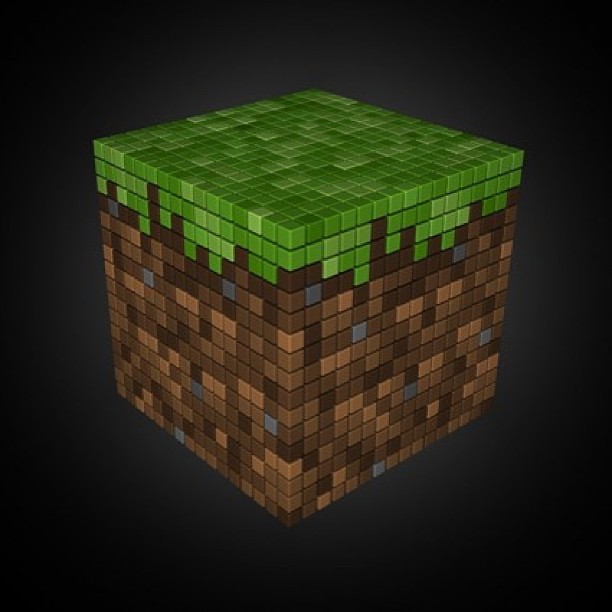The image is a detailed 3D computer model of a Minecraft dirt block with grass on top, set against a black background. The block appears to consist of hundreds of smaller cubes, creating a larger, cohesive structure. From the viewing angle, two sides and a portion of the top are visible, emphasizing the block's intricate construction. The bottom and sides predominantly feature various shades of brown, ranging from dark to light, interspersed with a few light blue cubes. The top consists of almost three complete layers, transitioning from a solid dark green and light green top layer to predominantly green layers with occasional flecks of brown. The entire block has a subtle glow, enhancing the distinct tiling of colors, and evokes the pixelated style iconic to Minecraft.